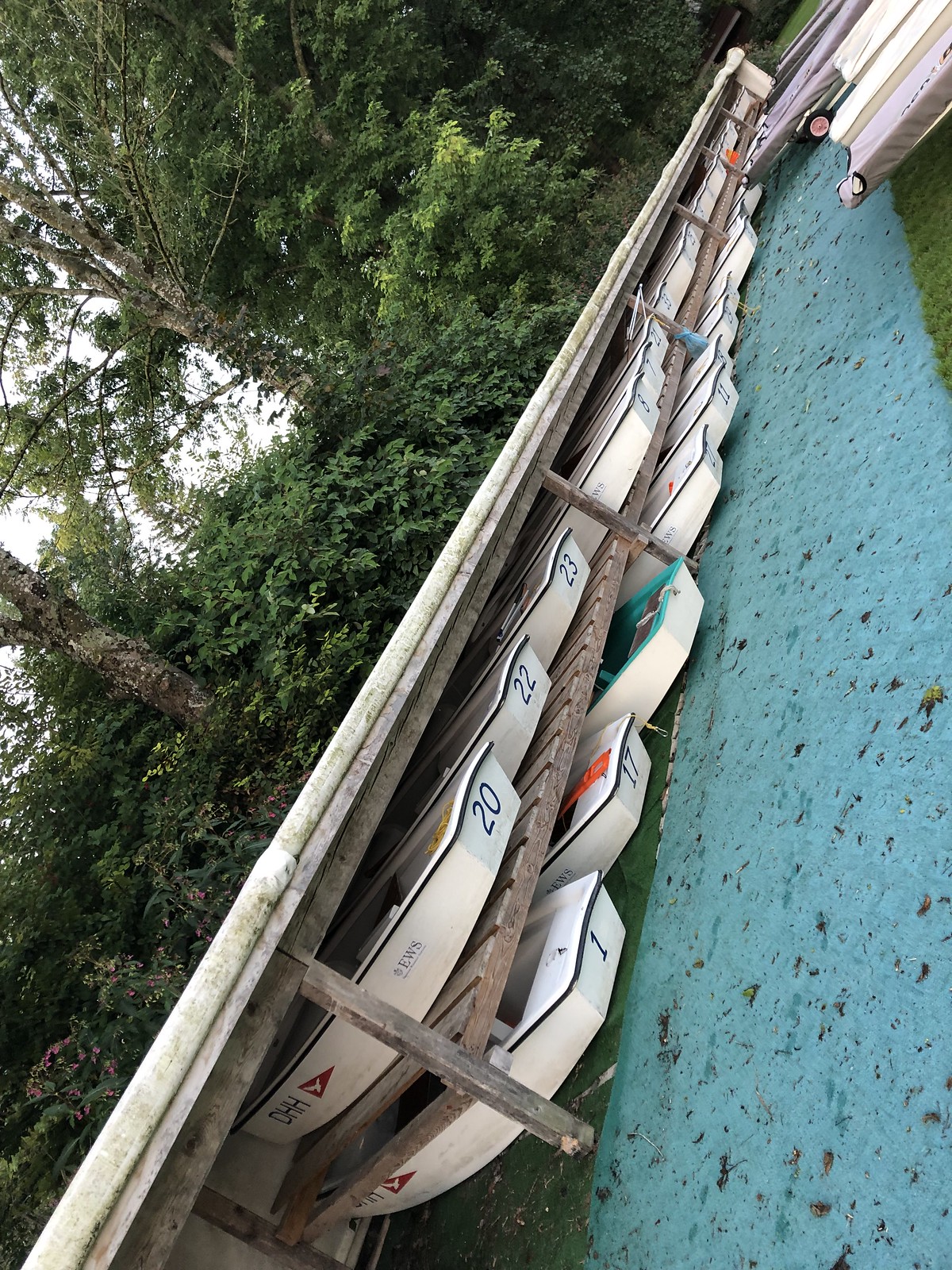This photograph, tilted to a vertical orientation, depicts a wooden storage area for small rowboats or dinghy-style boats. The storage consists of two layers of shelves made from pallets, with boats stacked two high. The white boats feature blue borders, numbers at the rear—ranging from 1 to 23—and markings including "DHH" alongside a red triangle containing a bird silhouette. The storage area is situated beside a grassy patch and dense green foliage, with bright green trees in the background. A speckled blue mat lies on the ground near the storage area, possibly used to slide the boats in and out. Additionally, there is a wagon nearby, likely used to transport the boats. The wooden structure shows signs of weathering, with some green algae on the PVC piping along its edges. The scene suggests a location near water, though the water itself is not visible in the image.